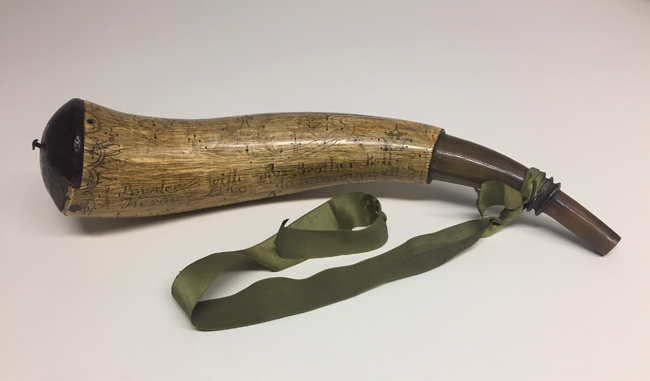This photograph features a historical artifact known as a powder horn, traditionally used during the pioneer period in the American West to carry black powder for reloading firearms. The horn itself, likely sourced from an animal such as a cow, is capped off at the wider end with what appears to be a wooden stopper, ensuring the container is sealed. On the opposite, narrower end, there's a spout designed for easy pouring of the powder. This particular powder horn is relatively plain, with minimal lettering and no elaborate engravings, distinguishing it from more decorative examples. Attached to the horn is an olive green cloth, presumably for securing it to a belt or another object. The artifact is set against an off-white, grayish rectangular background, with the wider part of the horn positioned to the left and the spout to the right. The simplicity and functional design of the horn, combined with its purposeful attachments, highlight its utilitarian role in historical firearm use.